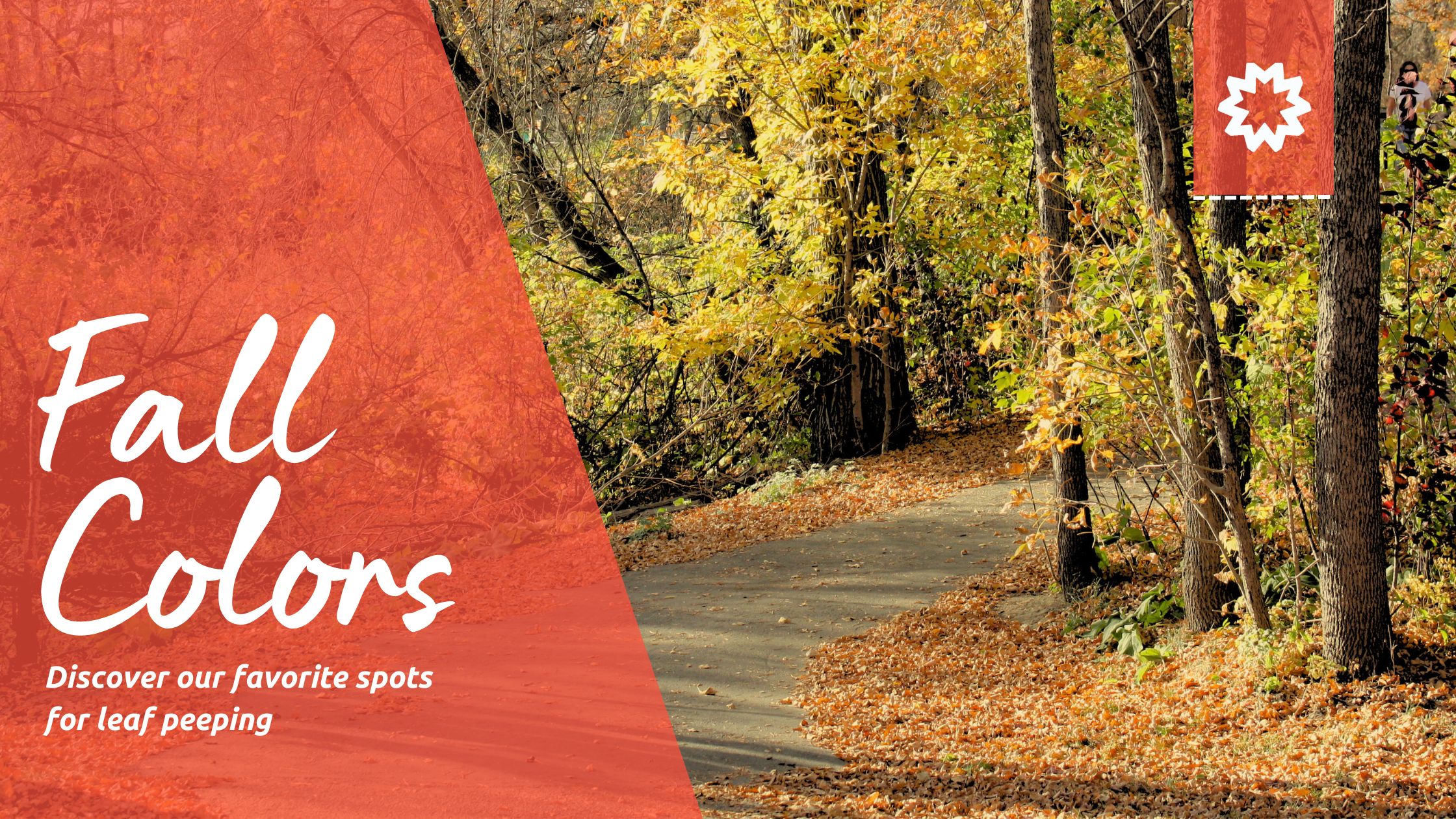The image is an advertisement promoting fall with a forest scene. On the left-hand side, a semi-transparent orange overlay displays the text "Fall Colors" in large white font, followed by "Discover our favorite spots for leaf peeping." The central focus is a picturesque pathway bordered by tall trees showcasing vibrant autumn foliage. The leaves exhibit a stunning array of yellow, orange, and remnants of green, indicative of the seasonal transition. The ground is scattered with fallen leaves, some forming small piles on either side of the gray path. A notable feature in the upper right-hand corner is an orange rectangle adorned with an intricate white star-like design. A subtle, possibly non-human figure wearing a gray shirt and black pants can be seen among the trees, adding an intriguing element to the scene. This inviting image captures the essence of fall, urging viewers to explore and enjoy the changing leaves.